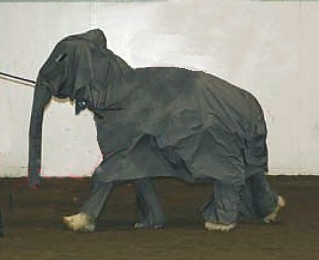The photograph depicts a side profile of what appears to be an elephant moving towards the left side of the frame, but it is actually a costume worn by two individuals, with distinguishable human legs visible. The costume is gray, complete with a long trunk, large ears, and cutouts for the eyes. The scene is set against a plain whitish-gray backdrop, creating a minimalistic environment. The floor beneath the elephant costume is brown, though it is not clear if it's dirt or carpet. Additionally, there's a gray rope pulling the costumed figures, reinforcing the costume illusion. The image captures this humorous and intriguing visual, evoking curiosity about the context of the scene.